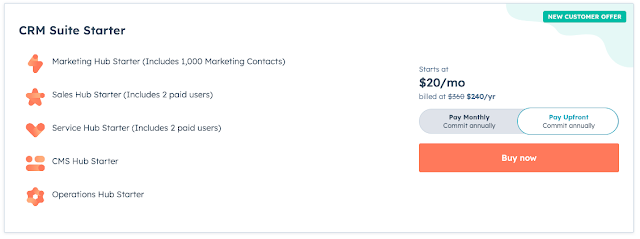The image is a horizontal rectangle with a very pale gray border around it and a white background inside the rectangle. In the upper left-hand corner, "CRM Suite Starter" is written in navy blue text. Beneath this title, there is a vertical list of options, each in navy blue text with a pale red icon to its left:

1. Marketing Hub Starter (includes 1,000 marketing contacts)
2. Sales Hub Starter (includes 2 paid users)
3. Service Hub Starter (includes 2 paid users)
4. Operations Hub Starter

In the upper right-hand corner, there is a wavy light blue section with a green box inside it that has "New Customer Offer" written in white.

Further down on the white background, it states that the price starts at $20 per month ("$20/mo"), billed annually at $240 ("$240/yr"). This information is also presented in navy blue text.

Beneath this, there is a slider bar with two options: "Pay Up Front" and "Commit Annually," which is highlighted in bright blue, and "Pay Monthly" and "Commit Annually," inside a gray bar.

At the bottom of the image, there is a red button with "Buy Now" written in white.